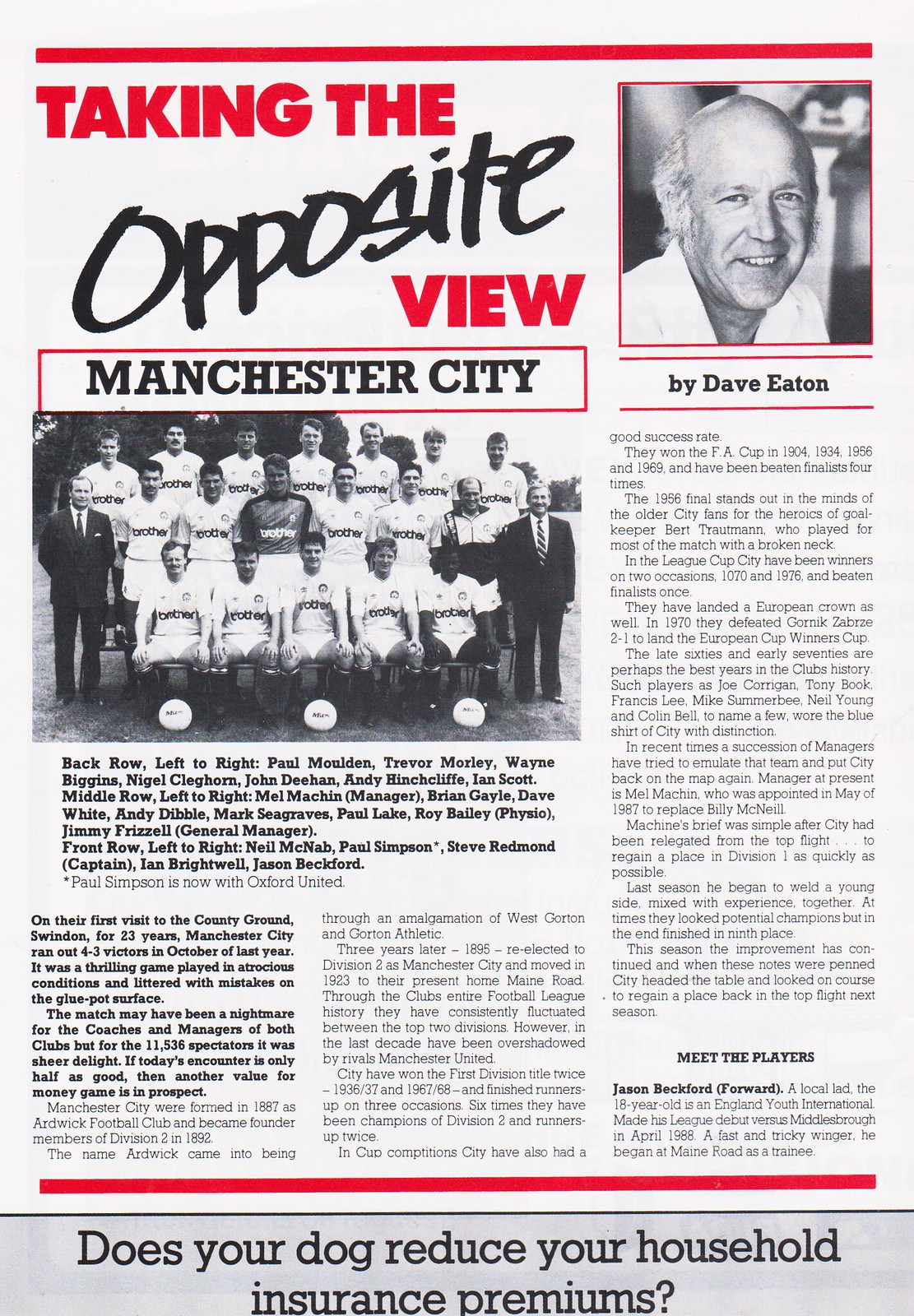The image depicts a page from a publication, likely a newspaper or a magazine, with a white background and predominantly black text, though some words appear in red for emphasis. At the top of the page, the headline reads "Taking the Opposite View," with "Taking the" and "View" in red, and "Opposite" in black. Below this headline, the text "Manchester City" appears in black, introducing the main subject of the feature.

Prominently positioned underneath this title is a black-and-white photograph of the Manchester City soccer team, arranged in three rows with the players donning white jerseys and shorts. The names of the players are listed beneath the photograph, arranged from left to right and back to front. On either end of the team photo, there are men in black suits, adding a distinguished touch to the formal team portrait.

On the upper right section of the page is a small black-and-white photograph of an older gentleman, presumably the author of the article. Directly below this photograph, the text "by Dave Eaton" confirms the author's identity. The article itself appears to be structured in three columns, delving into topics related to Manchester City.

At the very bottom of the page runs a gray bar with the intriguing question written in black: "Does your dog reduce your household insurance premiums?" This line adds an additional point of interest for the reader, contrasting with the main soccer-focused content.